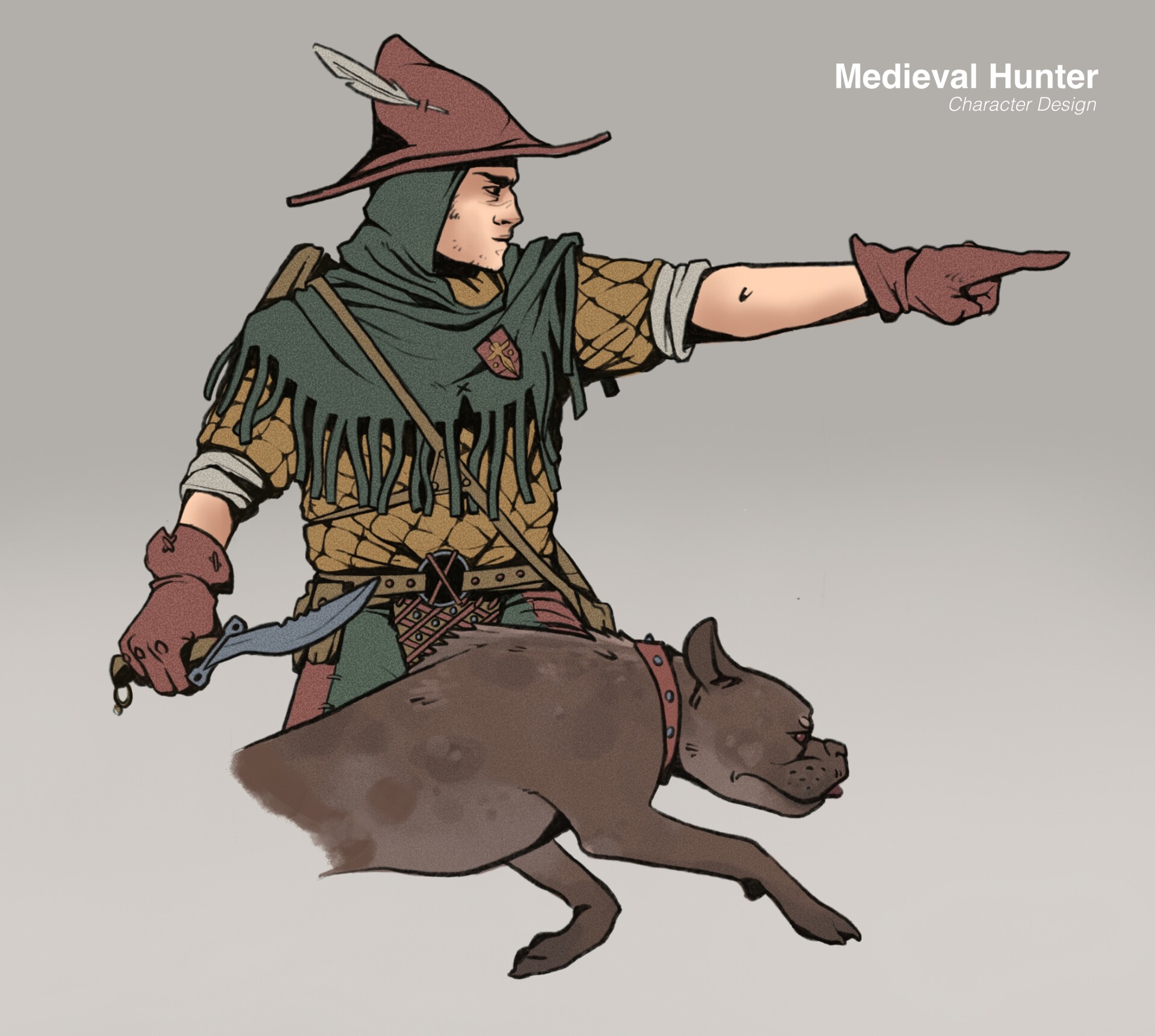The detailed image showcases a character design titled "Medieval Hunter," displayed in white lettering on a light gray background. The central figure is a cartoonish man dressed in medieval archer attire, distinguished by a red Robin Hood-style hat with a feather. He wears a green shawl, draping down over his leather armor, secured with a badge that features a red base and a golden sword. His ensemble includes a pair of red gloves, a headscarf of grayish dark green tint, and a satchel slung over his shoulder. He holds a large knife in his right hand at his side, while his left hand is outstretched, pointing forward with a determined scowl. Accompanying him is a brown dog with a red collar, energetically running towards the direction the man is pointing, embodying a sense of purpose and urgency. This illustration appears to be part of a character portfolio, fitting for a video game or tabletop RPG, emphasizing its dynamic and adventurous essence.